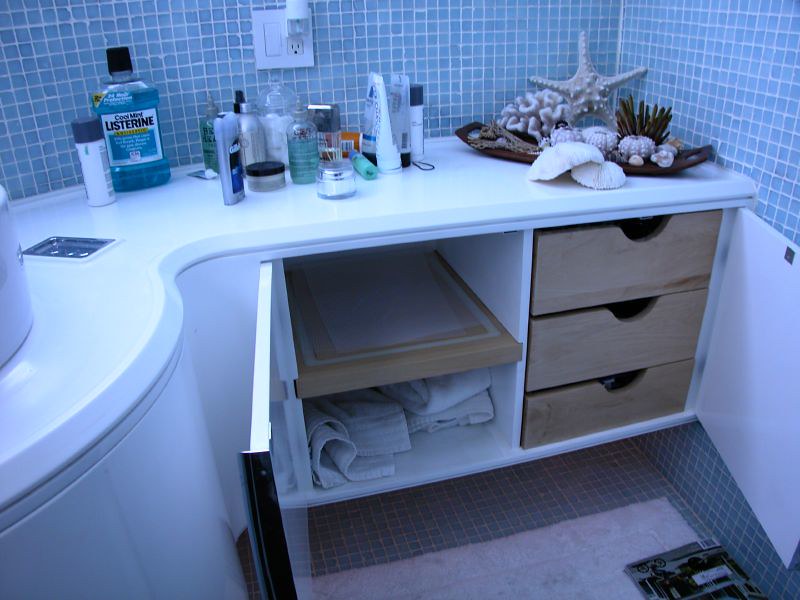The image portrays a detailed view of a bathroom countertop. The countertop itself is pristine white, while the cabinetry underneath appears to have a slight grayish or bluish hue. The countertop, sweeping from the right to the center of the image, is laden with a variety of bathroom essentials. Prominently positioned towards the left is a bottle of Cool Mint Listerine. Adjacent to it is a white canister with a black lid, though its label remains indistinguishable. Nearby, a container of what appears to be Gillette deodorant can be spotted amidst an assortment of other toiletries, likely including lotions and serums.

Above this collection of items, a power outlet equipped with a light switch is visible in the left center of the frame. The outlet has two sockets, the upper one occupied by an air freshener, while the lower socket remains unused. Dominating the rightmost section of the shelf, a decorative arrangement of sea-themed items, including an anemone and starfish, leans gracefully against the wall, adding a touch of coastal charm to the bathroom's ambiance.